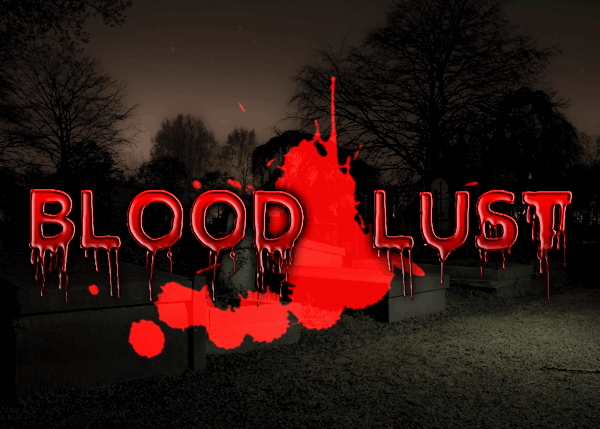In this nighttime image, the word "Bloodlust" is prominently displayed in the center in all-capital red letters, dripping like blood. Surrounding the text is an alarming blood splatter, with a massive splotch directly beneath the word. The background reveals a dimly-lit, outdoor setting, likely a park or cemetery, with grass and indistinct benches at the bottom, shadowy trees in the distance, and a dark, cloudy sky overhead. The colors of the scene are primarily black, gray, silver, tan, red, and green. The overall atmosphere is eerie and unsettling, hinting at themes linked to horror, possibly associated with a video game, movie, or company logo. The background details are obscured by the intense blood imagery, adding an element of mystery and terror.